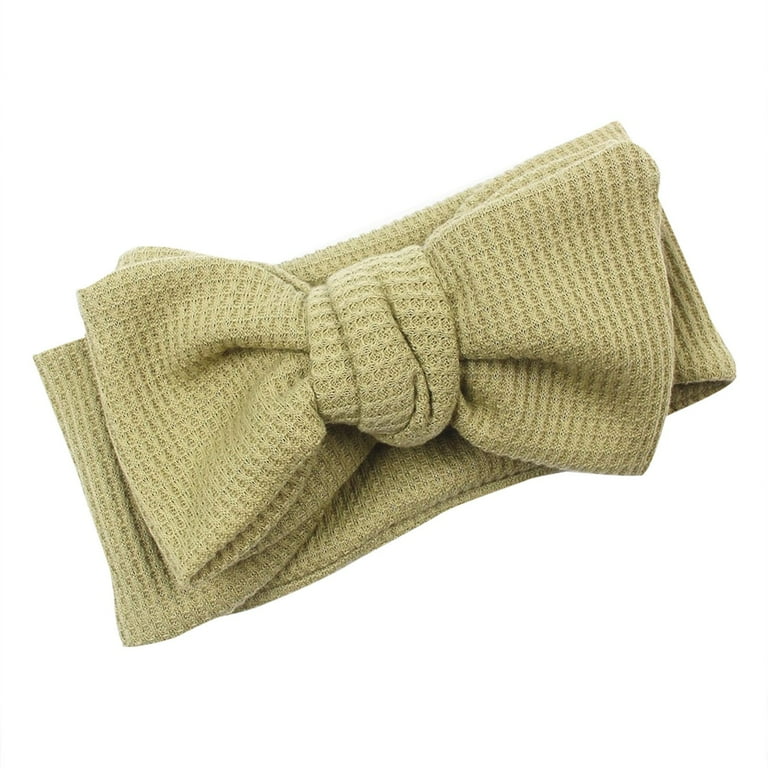The image showcases a light gray (or beige/tan) cotton head wrap that is textured and possibly stretchy, suitable for a young child. The highlight is a large, neatly tied bow prominently displayed at the front. The bow appears to be made of fabric loosely stitched or woven with thick thread, creating an evenly spaced pattern. It includes a central knot with a distinct crease extending downwards and slightly right, with another crease at the bottom turning left. The bow’s loops are fluffed out, almost as wide as the fabric piece beneath it, which lies completely flat. Both pieces are set against a solid white background, enhancing the simplicity and elegance of the design.